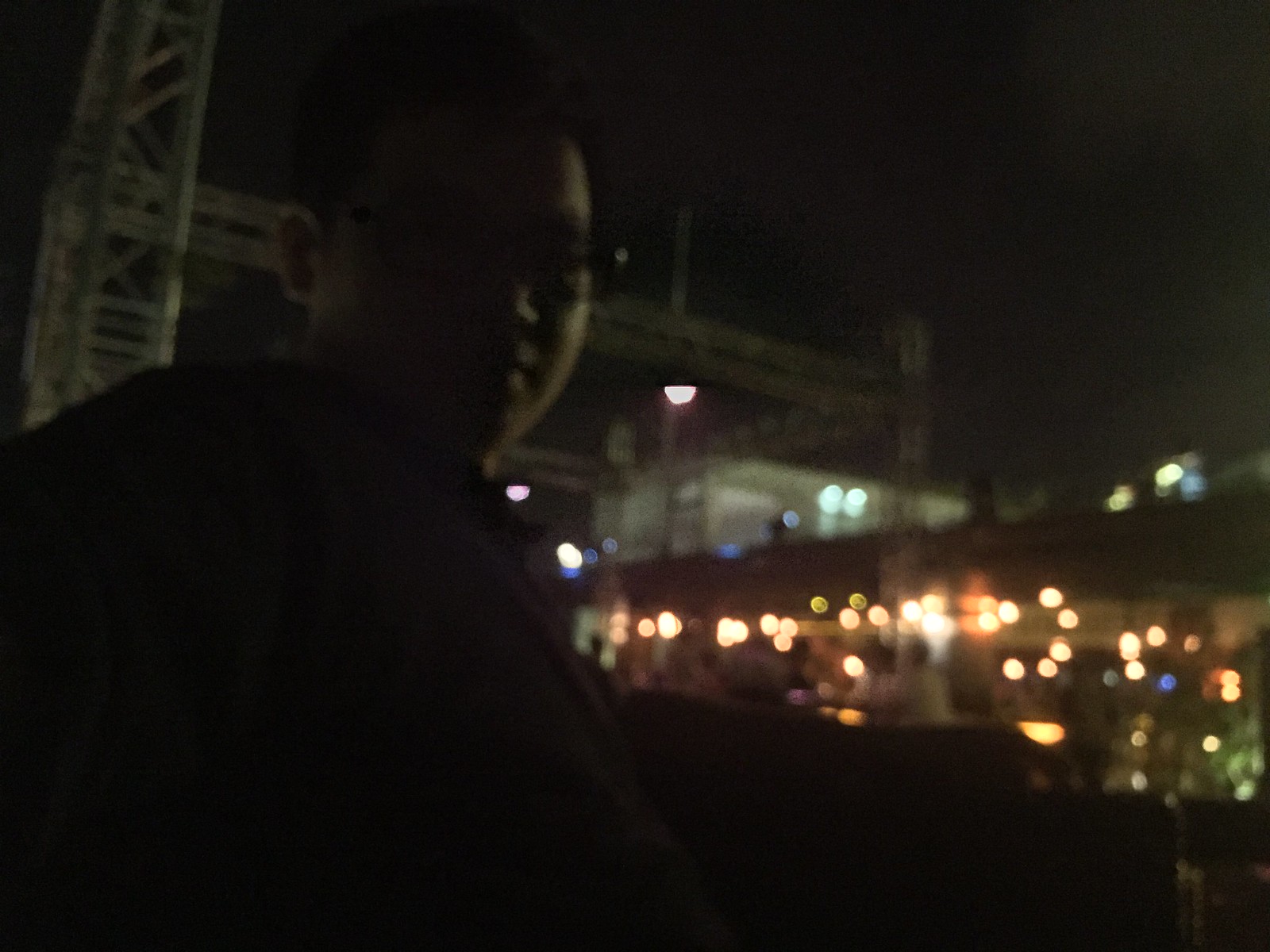In this nighttime cityscape, a blurry photograph captures a heavyset young man with dark hair and glasses standing in front of a towering building adorned with several lights. The image is notably dark, but a faint light illuminates the left side of his rounded face, revealing a pleasant expression. Behind him, a prominent metal framework adds to the urban atmosphere, while the background is aglow with a gradient of light, ranging from warm light orange to yellow and white hues. Despite the overall dimness and the man’s indistinct features, the city's vivid lights provide a hint of the bustling environment.